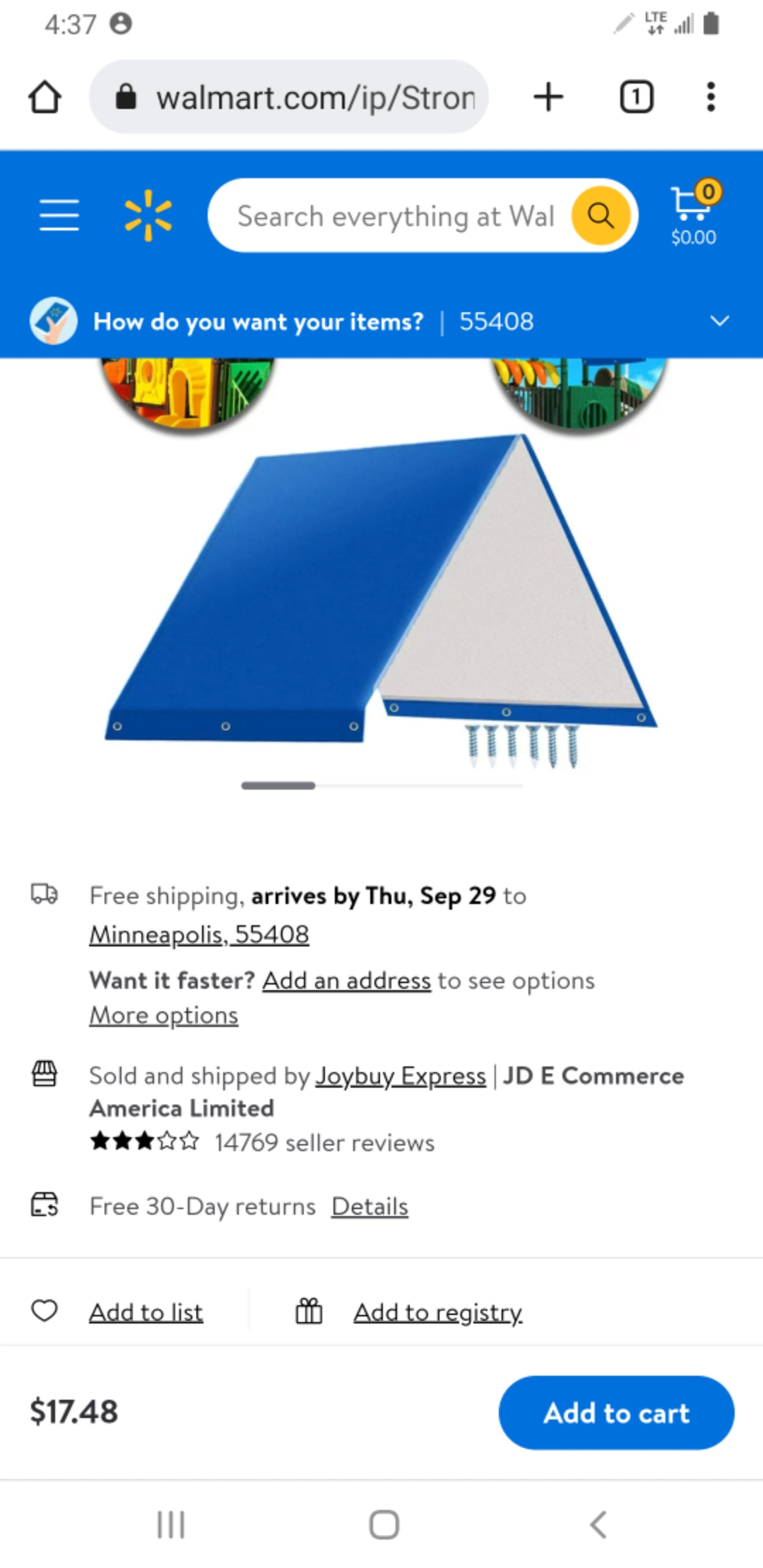This detailed caption provides a comprehensive description of a screenshot displayed on a cell phone, showing a webpage from Walmart.com.

---

The screenshot captures a webpage from Walmart.com displayed on a cell phone, providing a detailed overview of the site interface and the product information visible. At the top left corner, the time is shown as 4:37. Adjacent to the time is a home button. The webpage URL is partially visible as "walmart.com/IP/stron".

Just below the URL bar, to the left, is a search box with a plus sign outside it. There’s also a small square with the number "1" inside it, followed by three vertically stacked dots. Beneath this bar, the Walmart website's header is highlighted in blue, featuring a Walmart icon with three horizontal lines beside it, a search bar labeled "Search everything at Walmart", and a shopping cart icon showing a total of $0.00.

Under the header section, text prompts "How do you want your items?" followed by the zip code "55408". Below this text, there are two partially visible images. One resembles an upside-down and open blue folder with a white interior.

The text below the images reads:

- "Free shipping arrives by Thursday, September 29th to Minneapolis 55408. Want it faster? Add an address to see options."
- A "More options" link follows.
- "Sold and shipped by Joy Buy Express JD e-commerce America Limited," noted to have 14,769 reviews and a three-star rating.

Additional text indicates a free 30-day return policy with a "Details" link. Options for "Add to list" and "Add to registry" are available.

The current price of the item is $17.48, with an "Add to cart" button at the end.